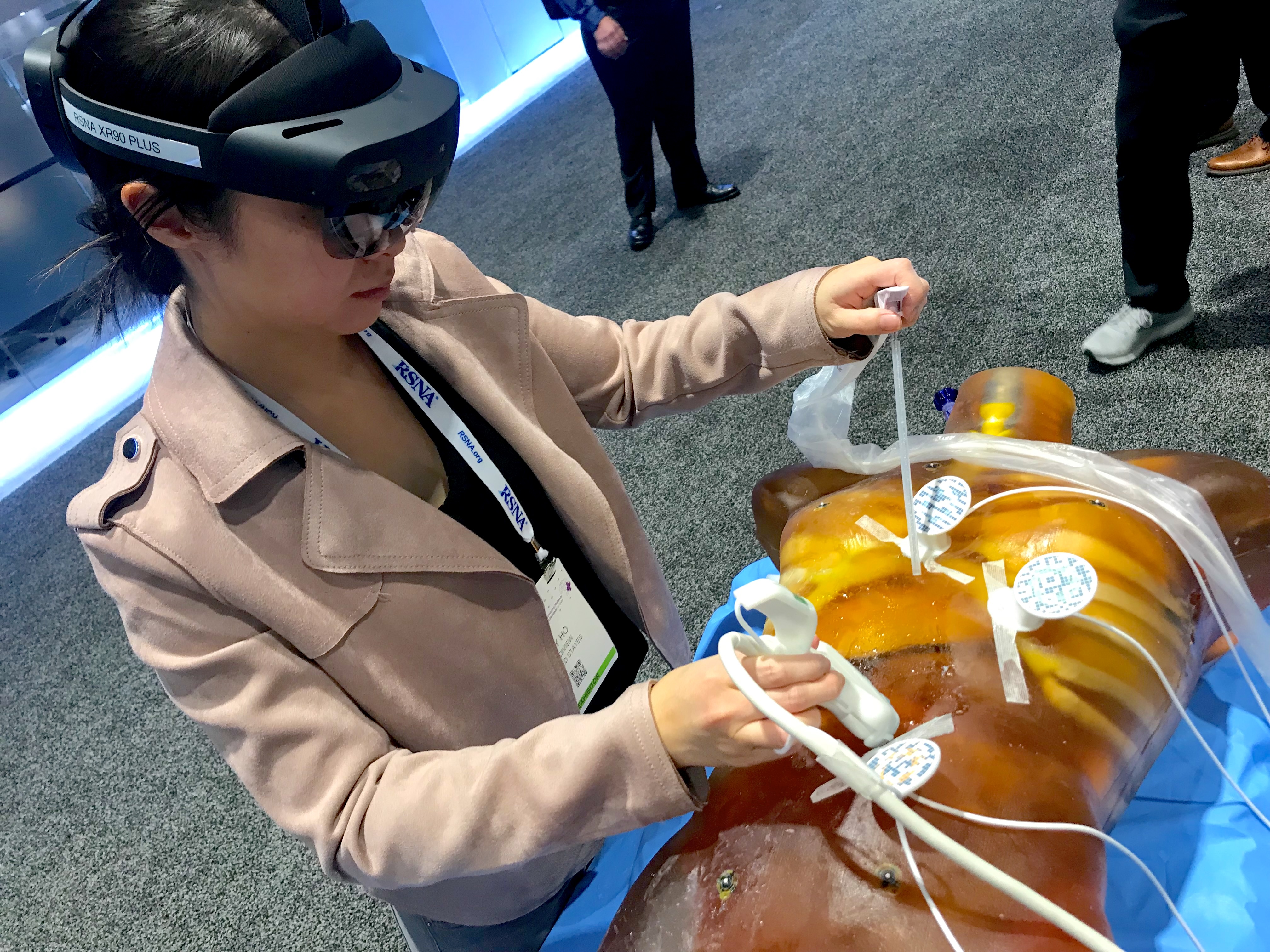The image portrays a woman, presumably a medical student or professional, engaged in a laparoscopic simulation. She is inside a well-lit environment, possibly a conference or training event. The woman is dressed in a brown jacket and a lanyard marked with "RSNK". Equipped with a VR headset or microscopy visor to enhance her vision, she meticulously operates using laparoscopic tools on a life-like dummy model made of silicon or plastic, simulating human organs. The dummy is positioned on a blue table. Observers can be seen in the background, indicating she is the focal point of a demonstration. The setting features a gray carpet, and other participants are visible, reinforcing the atmosphere of a busy and educational event.